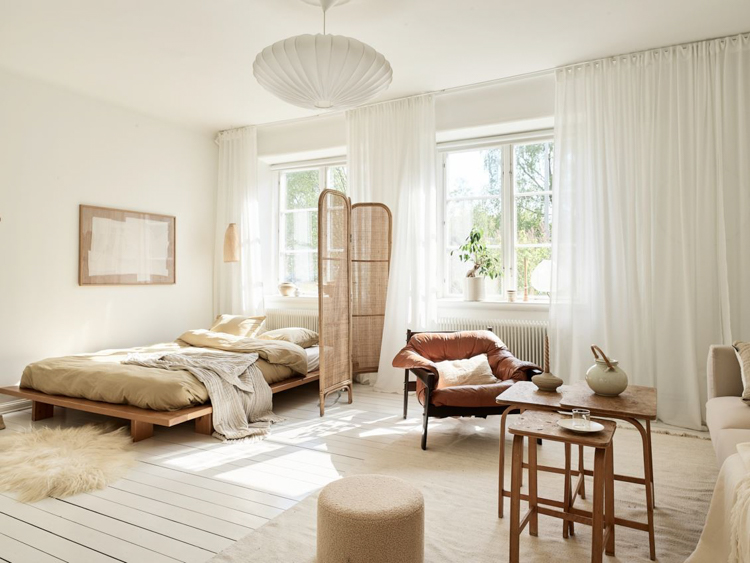This image captures a well-lit, spacious bedroom with a soft, cream and tan color palette that exudes tranquility. To the left, there is a low double bed made up with somewhat disheveled covers, lying on a wooden flat bed frame that may suggest a futon style. In front of the bed, a fluffy fur rug adds a touch of coziness to the white wooden floor. Adjacent to the bed is a bulletin board affixed to the white wall, adding a personalized touch to the space.

The center of the room features a comfortable chair with a pillow, and to the right, a sofa is positioned along with a table nestled between them. This table holds a teapot, a cup, and a dish, indicating a spot for relaxation and refreshment. The room is bathed in natural light pouring through two large windows adorned with floor-length, sheer white curtains, enhancing the room's airy feel.

A prominent globe bulb lamp with a shell-like design hangs from the ceiling, providing an additional light source. Behind the sofa, there is a framed painting that complements the room's aesthetic. Lastly, a wicker room divider is situated near the bed, adding texture and subtle separation within this serene living space.